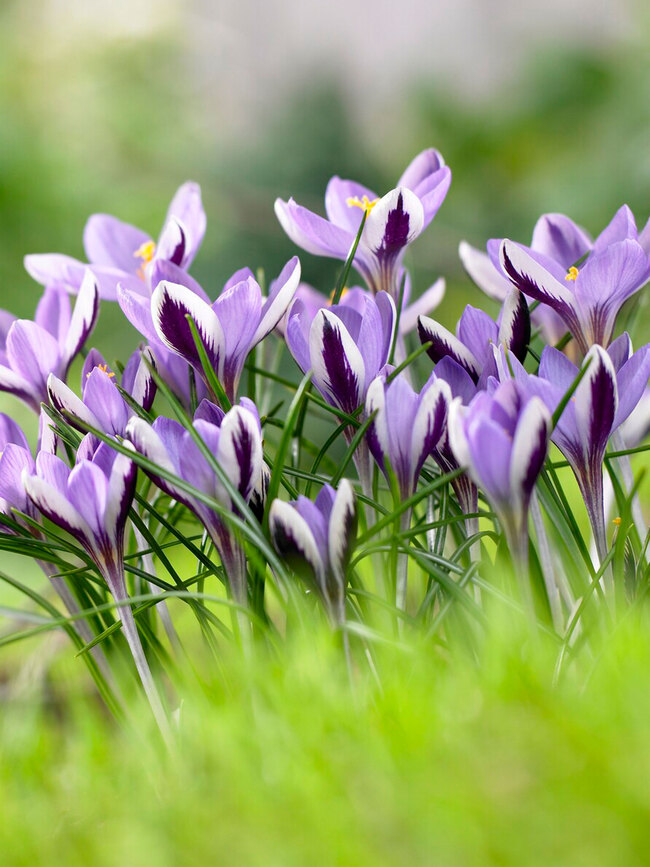This is a close-up, high-quality photograph of richly colored flowers blooming in their natural setting. The image sharply focuses on the flowers, showcasing their delicate petals that range from light lavender to deep purple, with some petals being white and adorned with dark purple centers. Each flower prominently features a vibrant yellow center, contrasting beautifully with their rich, bright green stems and leaves. Surrounding the flowers, there is a blurred background and foreground of greenery, with hints of grass blades at the bottom of the image and possibly trees or sky at the top. This blurring effect enhances the crispness and vividness of the flowers, making them stand out strikingly in the center of the photograph. The composition captures approximately a dozen flowers, some just beginning to open, set against the soft focus of their natural environment.